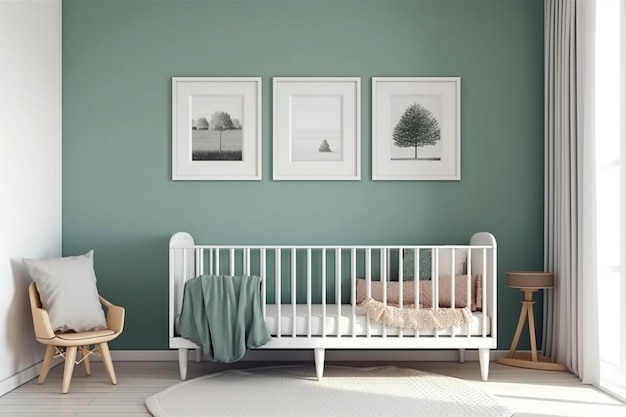The image depicts a modern nursery centered around a white crib with a white mattress, flanked by both a green wall and white walls on either side. The green wall behind the crib prominently features three equally spaced black and white framed photographs, each depicting trees. Inside the crib, there are several throw pillows, a green blanket, and some beige throw blankets, with a piece of lace hanging from the right side. To the left of the crib is a small beige chair with a gray throw pillow, and on the right side, there is a simple round table with two legs. A distinctive, elliptical-shaped white rug lies beneath the crib, contrasting with the gray wooden floors. The right-hand side of the image showcases tall white curtains over a floor-to-ceiling window, while a wooden decoration that resembles a tripod adds a subtle touch of rustic charm to the room.